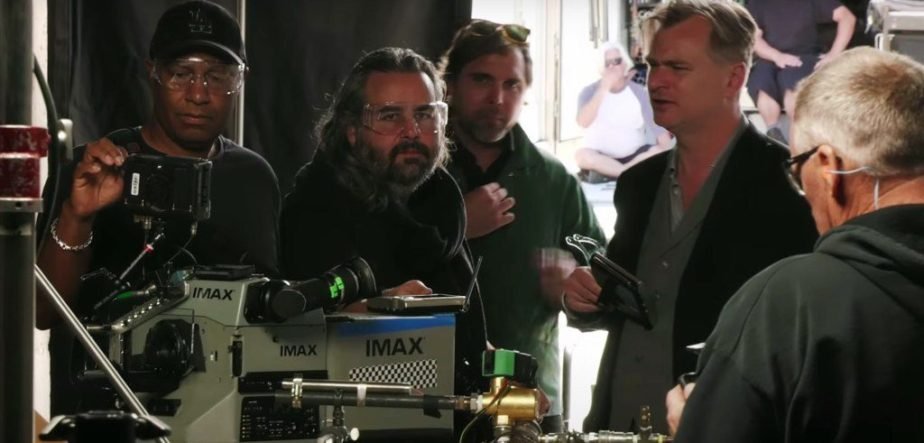The photograph features five men standing in an indoor room surrounded by various equipment. Prominently positioned in the lower left-hand corner is a substantial piece of chrome metal equipment branded with the word "IMAX" in large letters. Several lenses and attachments extend from this IMAX camera, suggesting an advanced setup for professional use. Two of the men on the left, who are wearing clear safety glasses, seem to be particularly hands-on with the equipment. One of them, wearing a black crew neck shirt and a baseball cap, is holding a small camera mount designed to hold either a smartphone or a small camera. To his right stands a bearded man in a black jacket, also wearing safety glasses, engaged in conversation.

Behind these two men, devices and lenses are arranged, culminating in one camera pointing toward the back of the photograph. In the central background area, the indistinct figure of a person with white hair and dark sunglasses can be seen, possibly supervising or observing the scene. Another man, positioned right-center and wearing a gray vest over a light shirt and dark jacket, holds an iPad in his right hand, suggesting he might be monitoring or controlling some aspect of the shoot.

In the lower right corner, we see the back of a man in a black hoodie with gray hair, who is also wearing glasses. The room has a professional yet bustling atmosphere, with people deeply engaged in a complex project, likely associated with IMAX and big-screen movie production.